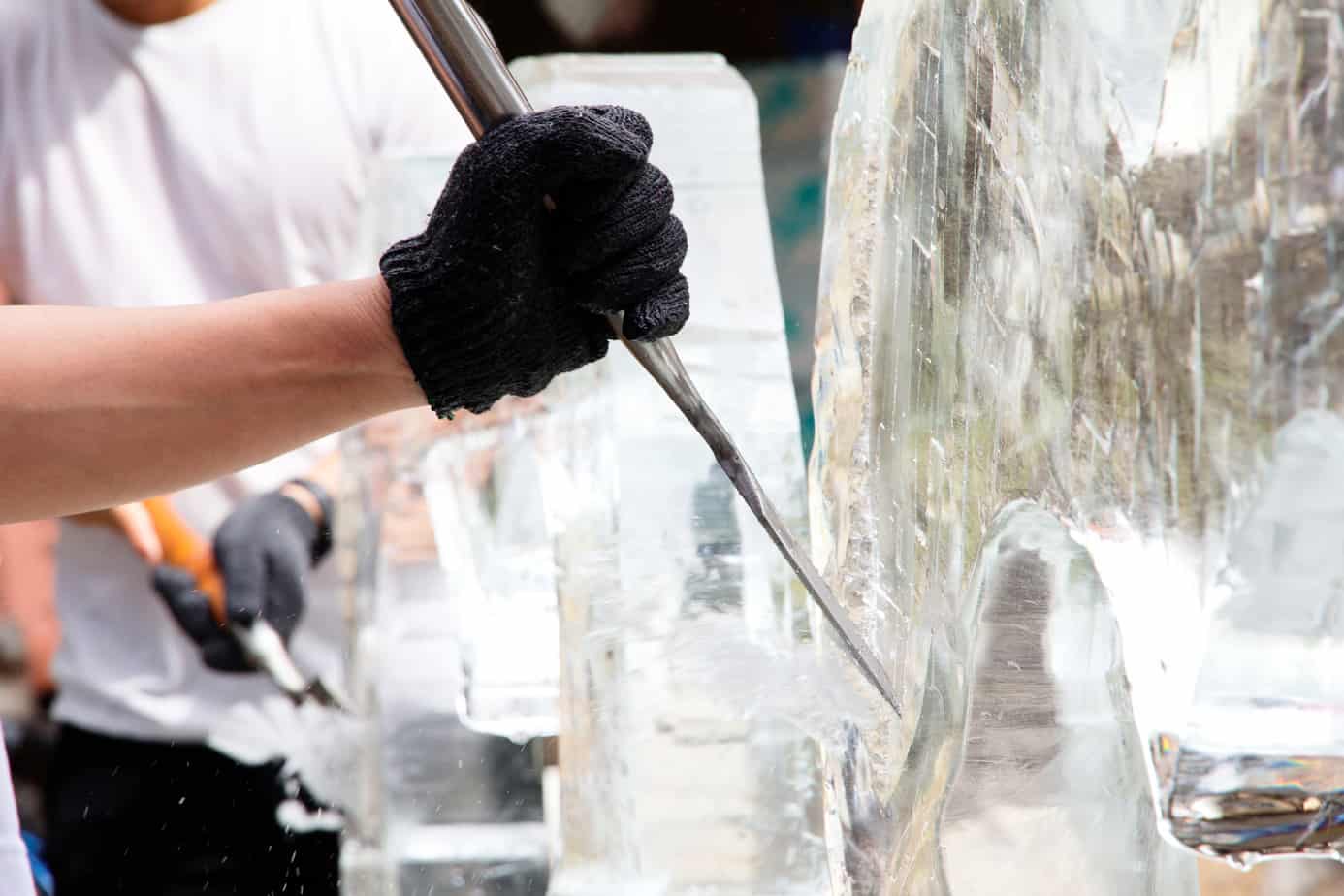The photograph features two people engaged in ice carving. Dominating the foreground on the right side of the image is a large, somewhat curved, scratchy block of ice reflecting a brownish hue, likely from its surroundings. It takes up roughly 40% of the image horizontally and extends vertically from bottom to top. A person, who appears Caucasian with a bare left arm donning a black glove, is shown chiseling away at the ice with a silver tool—resembling an ice pick with a flat, sharp end, angled at about 45 degrees. The glove, extending just an inch down the wrist, is gripping the metal tool tightly, with most of the tool out of view.

In the background, another individual, mostly blurred, is actively working on a different block of ice. This person is dressed in a white t-shirt and dark black pants, and his gloved hand is also seen handling a similar metallic tool. The ice blocks, both large and rugged in appearance, are in the initial stages of sculpting, exhibiting scratchy and chipped surfaces. The overall setting conveys a focused atmosphere of meticulous ice carving, capturing the intensity and precision of the work involved.